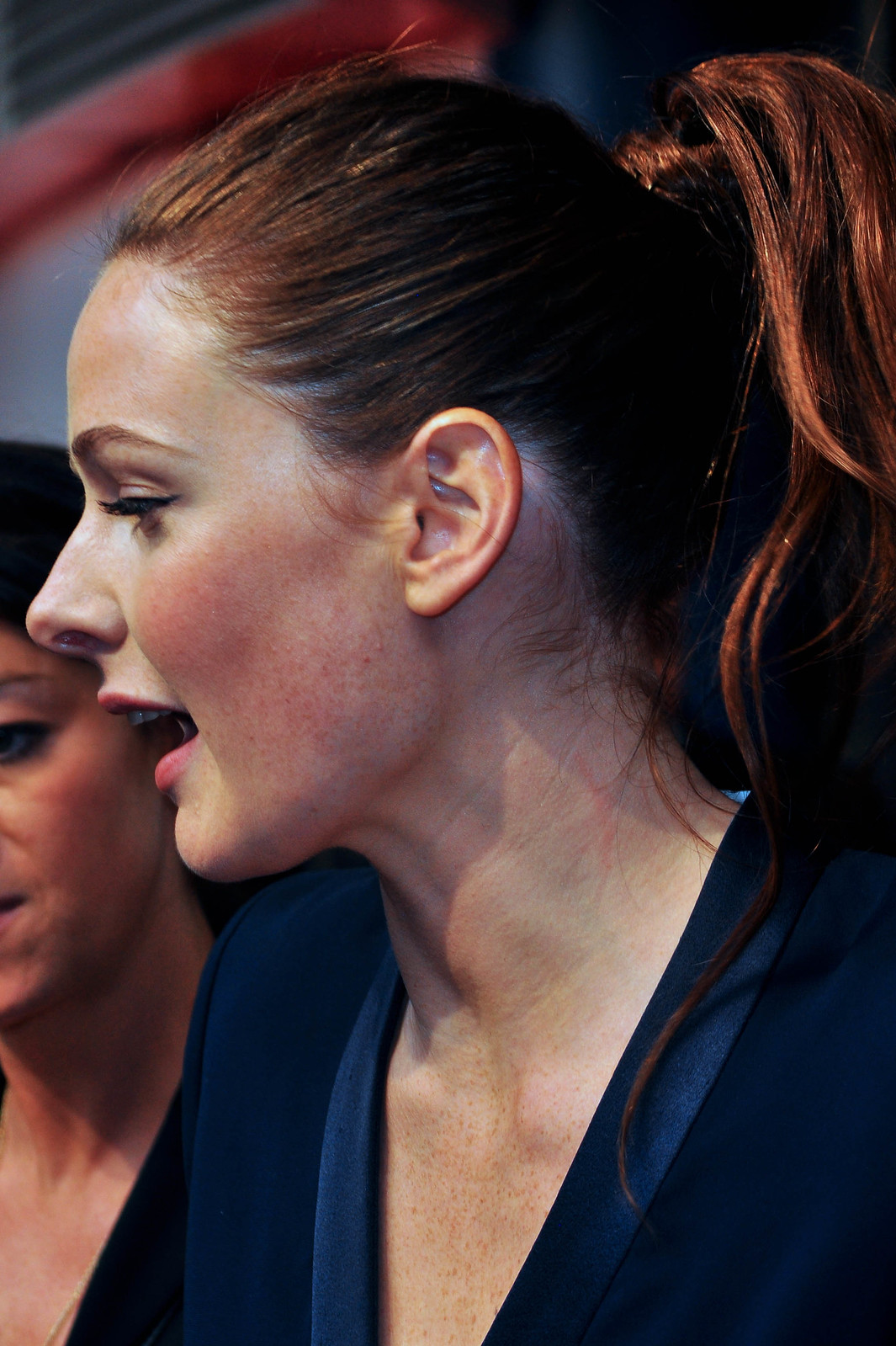This image depicts a close-up profile of a white woman with dark auburn hair, styled in an updo ponytail, showcasing her left side. She appears to be speaking, facing someone to her right. Dressed in a low v-neck blue blouse or dress, her attire reveals a small portion of her chest and possibly a white lining along the neckline. The background is intentionally blurred, featuring indistinct patches of white, red, and blue, contributing to the professional quality of the photograph. Another woman with dark black hair is partially visible behind her, although most of her features are outside the frame. The overall color scheme comprises shades of pink, red, peach, coppery reddish-brown, slightly greenish blue, black, white, gray, and silver. The main subject's light makeup and slender appearance enhance her poised and engaged expression within this professionally focused shot.